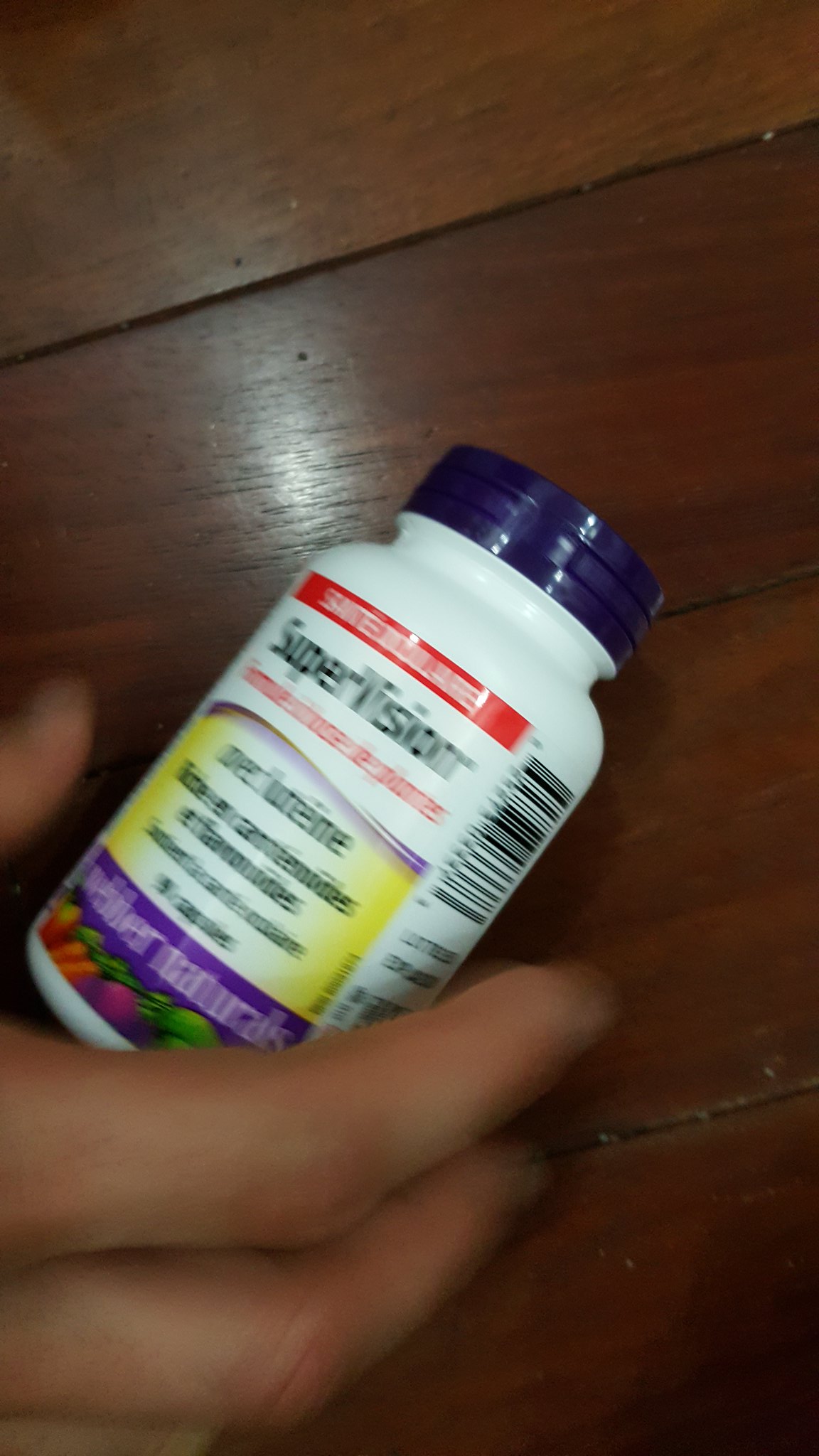This photograph showcases an extreme close-up of a brown wooden table, displaying the intricate texture and scratches of the wood, composed of parallel strips. In the foreground, a dark brown right hand is captured in motion, holding a small white bottle with a blue cap. The motion blur affects both the hand and the bottle, rendering detailed text on the label unreadable. However, the label prominently features the word "Supervision" in large black letters, followed by a red line and additional smaller text, including a purple banner at the bottom indicating "Weber Naturals". The lower part of the label displays colorful images of various vegetables and fruits. A barcode is visible on the right side of the bottle, adding to the overall detail of the scene.